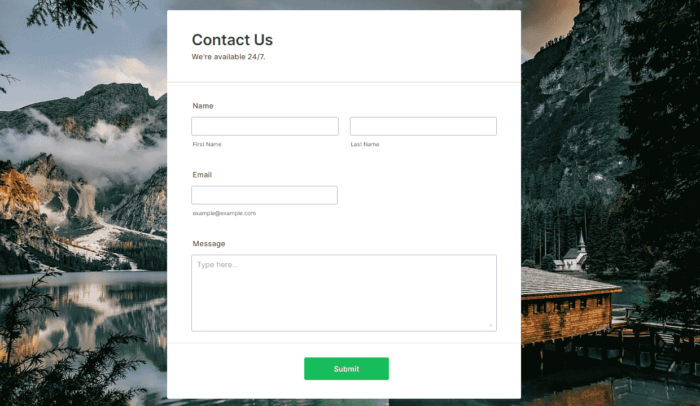A visually striking image features the "Contact Us" page displayed on a computer screen, overlaying a breathtaking wintry mountain landscape. The background reveals snow-capped mountains, extending down to the lower slopes, indicating a wintry season. Mist and fog shroud the middle sections of the mountains, creating an ethereal atmosphere, while wispy white clouds float in the blue sky at the top left corner. Contrastingly, darker gray clouds loom toward the right, adding depth to the scene. 

Nestled within this picturesque setting, a small white church and a rustic wooden cabin can be seen on the right side of the image, enhancing the serene, natural beauty.

In the foreground, the contact us page is prominently displayed with a clean, white background. The header reads "Contact Us," followed by the text "We're available 24/7." A subtle gray line extends horizontally, sectioning the page neatly. Below, user input fields are presented: boxes labeled "First Name" and "Last Name" are positioned side by side, followed by an "Email" field and a larger message box below it. At the very bottom, a green "Submit" button is ready for use. The juxtaposition of technology with nature highlights a harmonious blend of modern convenience and timeless beauty.